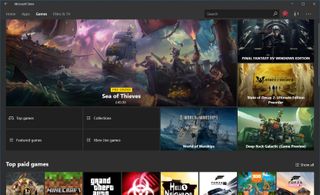This small screenshot showcases the interface of a gaming app, likely an online store. Dominating the upper left portion, an image featuring the game "Sea of Thieves" occupies three-quarters of the screen width and almost half of its vertical space. The vibrant scene depicts pirates navigating tumultuous seas under blue and purple skies, engaging in battles with pistols on antique ships.

To the right, there are smaller screenshots of other games, although their titles are not discernible. Beneath the "Sea of Thieves" image, a grid of four grey options — possibly representing user collections or purchase options — is displayed. Below these, the store highlights the "Top Paid Games," listing eight game icons. Among them, recognizable titles include "Minecraft," "Grand Theft Auto," and a game related to "Biohazard," with the rest being unclear.

The app's background is grey, and the store's specific branding or platform remains unidentified, though it could be a marketplace for Xbox, Steam, or another gaming service.